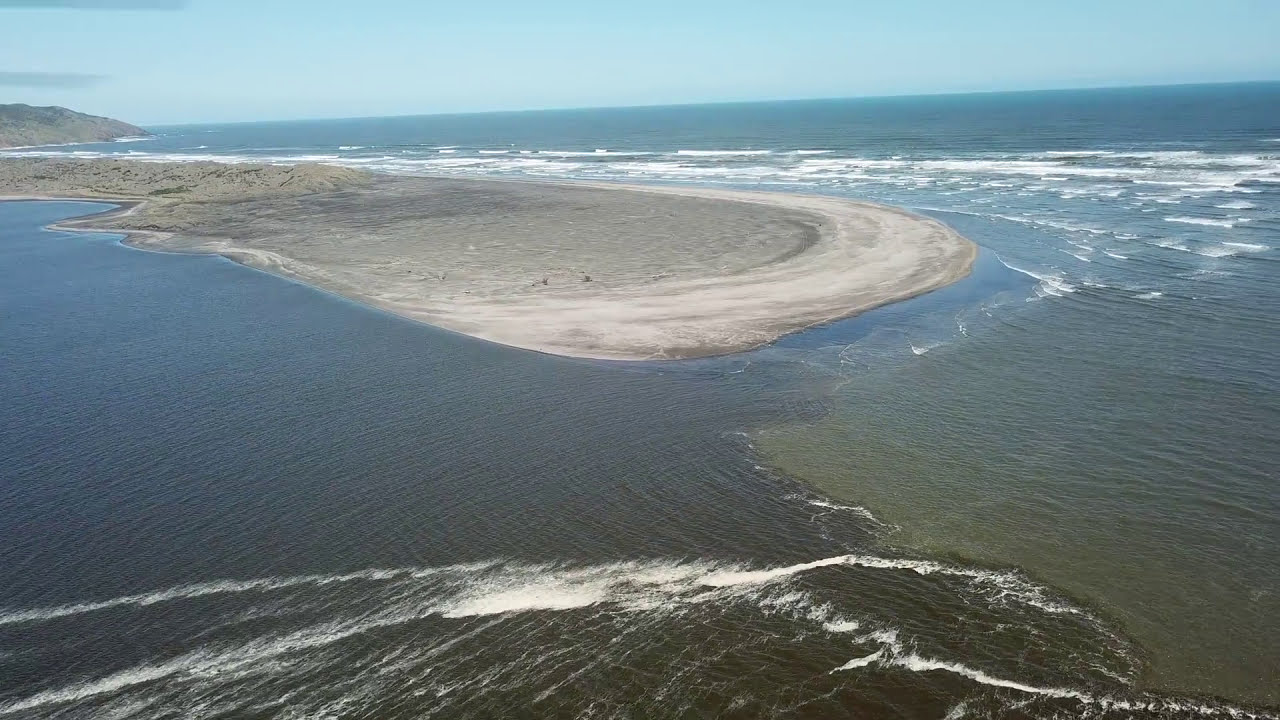This photograph captures a scenic view of the sea from an elevated vantage point. Dominating the center is a mostly flat, light brown island of irregular shape, surrounded by swirling waters. The sea itself displays a gradient of blues and greens, punctuated by whitecaps and waves, creating a lively and dynamic appearance. On the far left, another island with higher elevation and a potential cliff or small mountain adds depth to the scene. The lower half of the image is primarily water, while a sandy outcropping stretches into view from the bottom, leading to the central island. The sky above is a clear, light blue with few clouds, enhancing the overall tranquility of the setting. The water appears exceptionally clear, revealing possible sandy patches beneath, and the untouched, pristine quality of the central island suggests a serene, unspoiled environment.